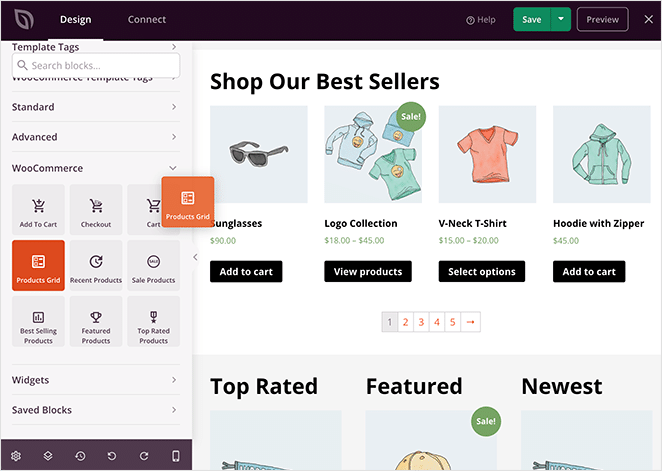This image is a detailed screenshot of a clothing and accessory website. In the upper left-hand corner, the brand logo, a minimalist leaf design, is prominently displayed. Adjacent to the logo are two navigational tabs labeled "Design" and "Connect." The screenshot shows that the user is currently on the "Design" tab.

Moving to the upper right section, there is a help button represented by a question mark, followed by a green "Save" button with an optional drop-down menu, and a "Preview" button accompanied by an 'X' symbol.

On the left-hand side, the interface features a label "Template Tags" above a search bar with placeholder text that reads "Search Blocks...". It appears that part of the text is obscured by the search bar. Beneath this, there are toggles for "Standard," "Advanced," and "WooCommerce" options.

Displayed below these toggles is a grid-like arrangement of buttons, each marked with symbols for various functions: Add to Cart, Checkout, Cart, Products Card, Recent Products, Sale Products, Best-Selling Products, Featured Products, and Top-Rated Products. The "Products Grid" button is highlighted in orange, indicating its selection. Additional tabs, such as "Widgets" and "Saved Blocks," are located lower in this section, along with functional buttons including "Edit," "Undo," "Redo," and more.

On the right-hand panel, large text reading "Shop our Best Sellers" leads the content. Listed underneath are featured items: Sunglasses, Logo Collection, V-Neck T-Shirt, and Hoodie with Zipper, each displaying various price points and action buttons for "Add to Cart," "View Products," and "Select Options."

The bottom part of the panel shows pagination with five visible numbers and an arrow button for navigating through pages of products. Finally, there are three sections labeled "Top-Rated," "Featured," and "Newest," each partially displaying products beneath them, suggesting further selections beyond the visible frame.